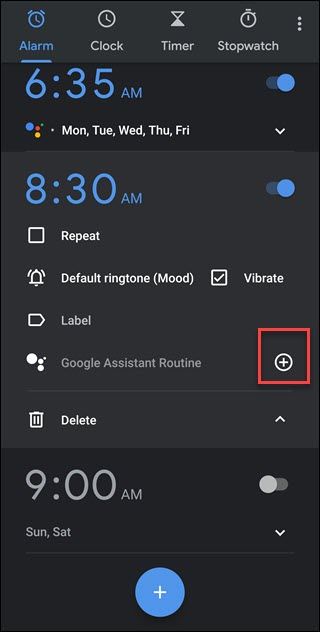The image is a screenshot of a clock application interface displaying various time-related functions, including an alarm, clock, timer, and stopwatch, organized within a menu. The alarm section shows two set alarms: one for 6:35 AM, active on Monday, Tuesday, Wednesday, Thursday, and Friday, and another for 8:30 AM, with no repeat activated. The alarm settings indicate that the default ringtone will be used and vibration is enabled. Additionally, there is a Google Assistant routine highlighted in red, scheduled for 9:00 AM on Sundays and Saturdays, though it is not enabled. At the bottom of the interface, there is a prominent "add" button. The background features shades of black and grey, while other interface elements are accented in blue and white.